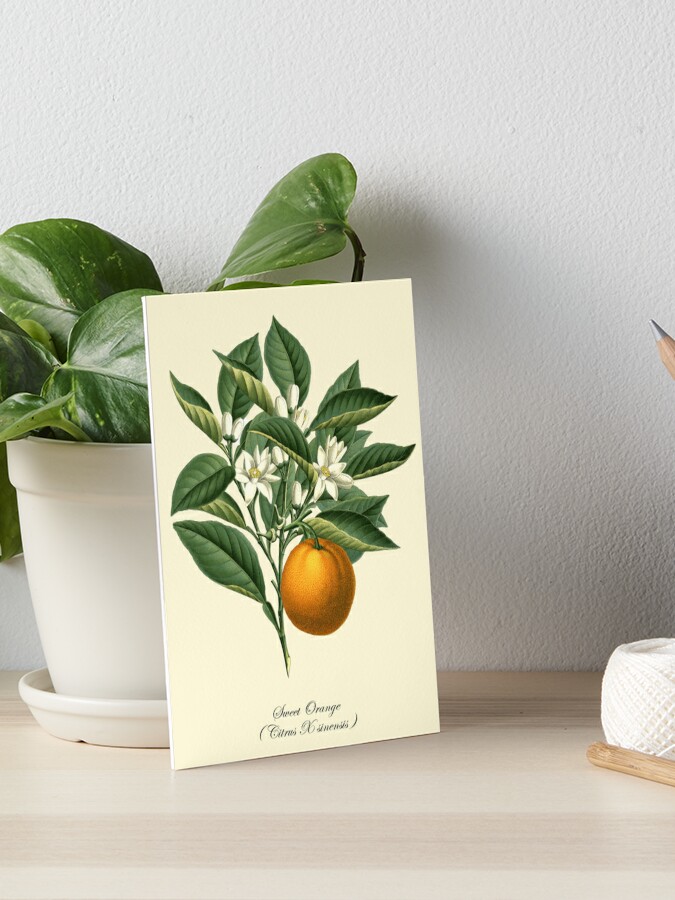In the image, a hand-drawn card depicting a "Sweet Orange" branch rests against a light tan pot on a wooden tabletop. The pot contains a plant with green leaves, positioned off-center to the left on the tabletop, which has a subtle wooden texture. The card, featuring a detailed illustration of an orange branch with lush green leaves, white blooming flowers, and a single vibrant orange fruit, is labeled with "Sweet Orange" and the Latin names of the orange variety beneath it. The background consists of a plain white wall, contrasting with the green foliage and the light tones of the wooden tabletop and pot. To the right of the pot, a spool of white yarn and a metallic silver pencil tip are visible, adding small yet distinct details to the setting.